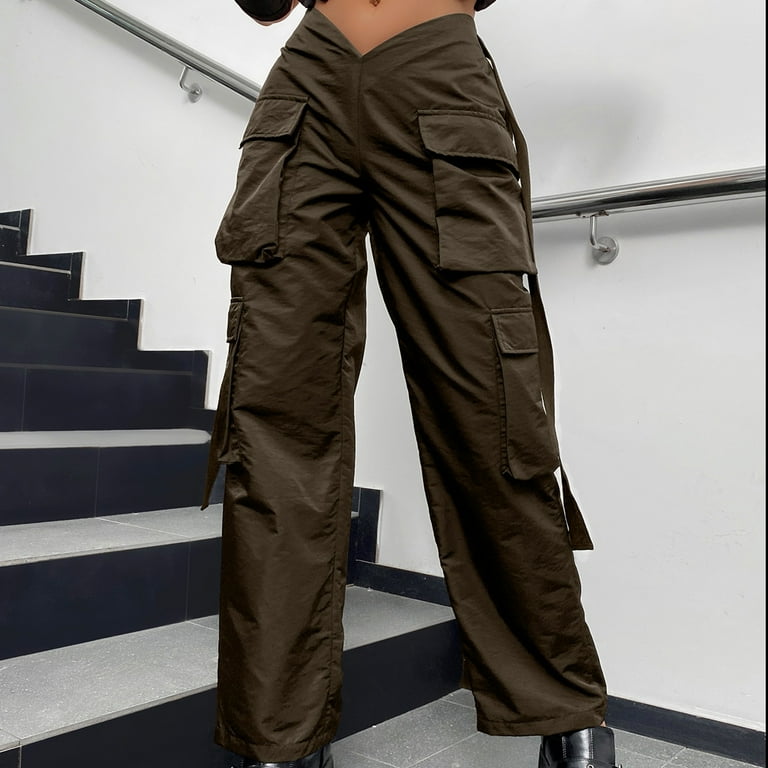In this image, a young woman stands at the bottom of a stairwell, where stairs ascend towards a higher level. The stairwell features a silver handrail and steps with dark gray and light gray, or black and white, tiles. The walls of the stairwell are white. The foreground of the image prominently displays the woman's lower torso to her feet. She is dressed in olive drab cargo pants with multiple pockets — two near the waist and two at the knee area. The pants have a distinctive V-shaped waistline and a long, untied belt draped down. The woman’s midriff, specifically her belly button, is visible, suggesting she is wearing a crop top. Her black leather shoes are partially visible, revealing just the top portions. The floor she stands on features gray and blue tiles, completing the detailed scene.